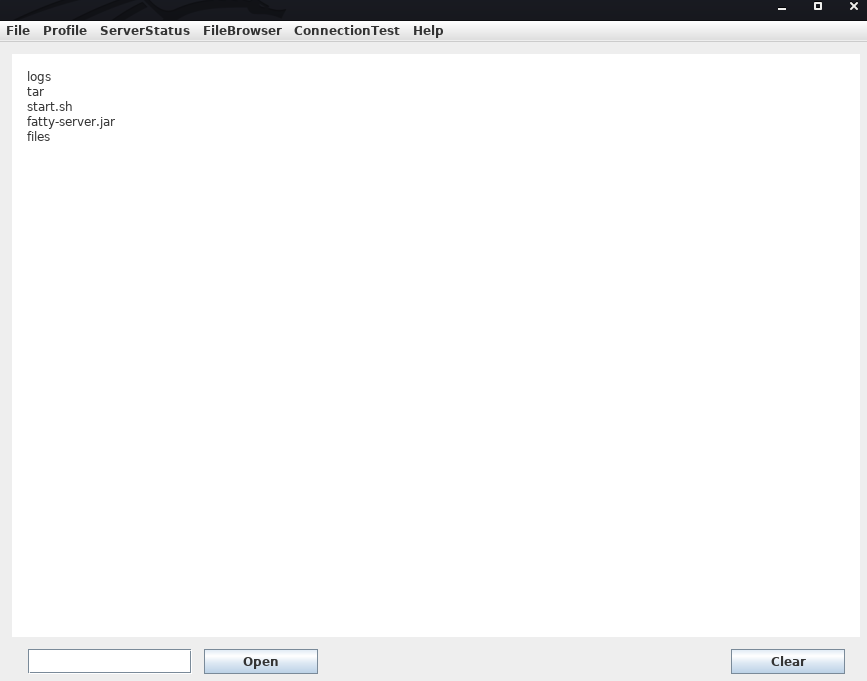The image depicts a streamlined settings or file management page for a website. The page features a black border along its top edge, housing three control buttons: minimize, full-screen view, and close. 

Beneath this border, there are several tabs labeled "File," "Profile," "Server Status," "File Browser," "Connection Test," and "Help." The primary area of the page is predominantly white, interspersed with a few black text entries arranged vertically. These entries include "logs," "tar," "start.sh," "fattyserver.jar," and "files."

At the bottom left corner of the page, a search box is situated, flanked by a button presumably intended for file opening, and a clear button to reset the search. The overall design is minimalistic, focusing on the essential elements with little visual embellishment, making it easy to navigate and functional.